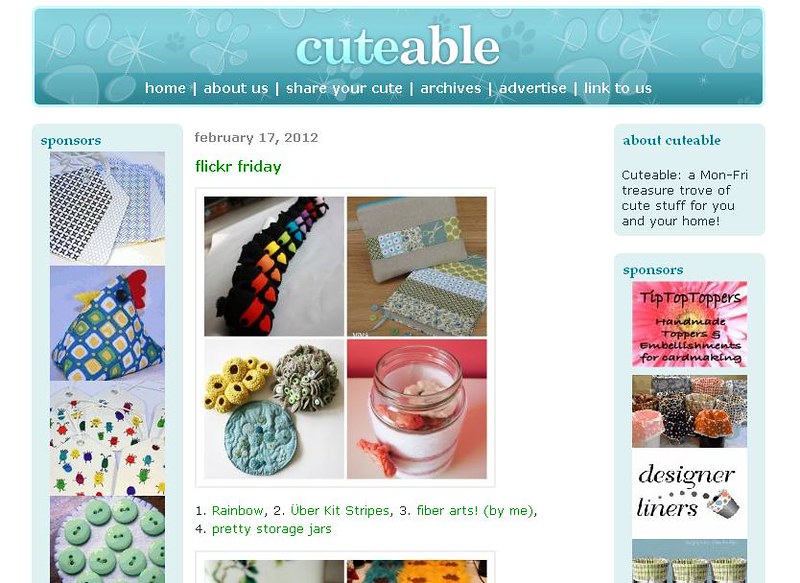This screenshot captures the homepage of a website titled "Cuteable," presented with a blue background and adorned with shimmering dog and cat paw prints. At the top, the site name is clearly displayed, with "Cute" in light blue and "able" in white. Beneath this, a navigation menu offers links to Home, About Us, Share Your Cute, Archives, Advertise, and Link to Us. The current post is dated February 17, 2012, and is titled 'Flickr Friday.' Below this, a 2x2 grid showcases various art projects: a candle in a mason jar, a pillow, and other cute crafts accompanied by a label reading: 1. Rainbow, 2. Uber Kit Stripes, 3. Fiber Arts, Buy Me, 4. Pretty Storage Jars. Flanking the main content, there are banner ads labeled 'Sponsors' featuring 'Tip Top Toppers' and 'Designer Liners.' Additionally, a section in the top right corner provides a brief description: "Cuteable, a Monday through Friday treasure trove of cute stuff for you and your home."